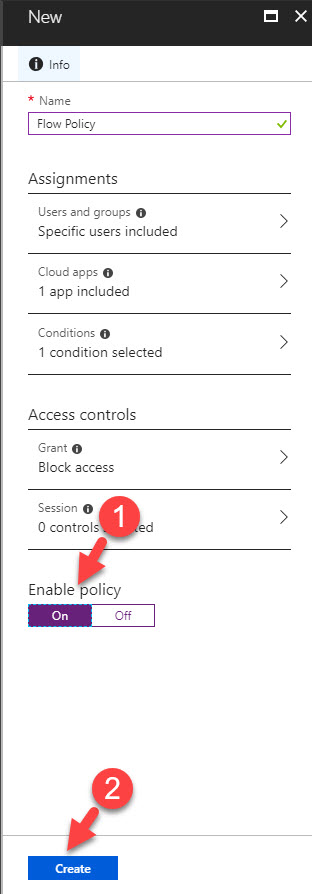This screenshot likely captures a section of a software interface, possibly on a tablet or a computer screen. The interface is designed for configuring some sort of flow policy or security settings.

At the very top, there is a black bar labeled "New" with an icon to the left and an X button to the right, suggesting a new configuration is being created. Immediately below this bar is a section titled "Info" and under it, a required field labeled "Name" indicated by a red asterisk (*). Adjacent to the "Name" box is a green checkmark symbol next to the text "Flow Policy".

Below this "Info" section is the "Assignments" section, consisting of three subsections:
1. **Users and Groups**: This subsection includes a small eye icon inside a black circle, indicating visibility or confidentiality settings. It states "Specific users included" with a right-facing caret (>), implying additional settings available on a subsequent screen.
2. **Cloud Apps**: Similar to the first subsection, it has an eye icon in a black circle, with text indicating that “1 app included" and a right-facing caret.
3. **Conditions**: This has an eye icon in a black circle as well, mentioning "1 condition selected" with a corresponding right-facing caret.

Following these, there is a section labeled "Access Controls" that is divided further into two categories:
- **Grant**: Accompanied by an eye icon in a black circle and text saying "Block access" with a right-facing caret.
- **Session**: Featuring an eye icon in a black circle, and the text "Zero controls ...", though the rest of the text is obscured by a red circle displaying the number one (1).

The last notable section is titled "Enable Policy," with an option to toggle the policy between "On" (highlighted in purple) and "Off" (highlighted in white).

Finally, a red circle marked with the number two (2) and an arrow points towards a bar labeled "Create," indicating the final step to create or save the policy configuration.